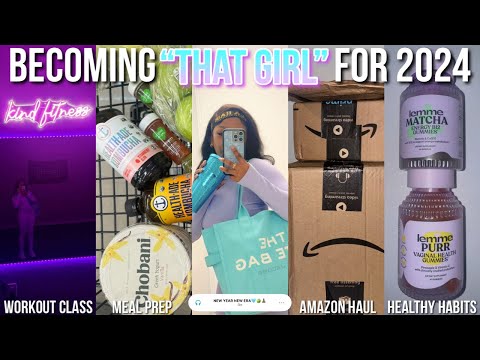This image is an advertisement with a grid layout, divided into five vertical columns against a backdrop of black horizontal bars. At the top, bold text in white reads "Becoming That Girl for 2024," with "that girl" highlighted in a gradient from blue to purple. Each column features a distinct thematic photograph and a label at the bottom in white text, indicating different aspects of a self-improvement routine. 

The first column shows a black woman at a gym, taking a selfie in front of a mirror with a purple neon sign that says "Kind Fitness." This column is labeled "Workout Class." 

The second column captures various meal prep ingredients in a shopping cart, including Chobani yogurt, vegetables, and bottles, labeled "Meal Prep."

The third column features a black woman dressed in a purple outfit with a blue bag, sipping from a blue tumbler while taking a selfie, though the label at the bottom is obscured.

The fourth column displays two brown Amazon boxes stacked on each other, plainly labeled "Amazon Haul."

The fifth and final column contains two bottles of gummy vitamins from Lemmy, labeled "Healthy Habits." The vitamins are specified for vaginal health and energy.

Each image contributes to a cohesive narrative illustrating the steps to "becoming that girl" in 2024 through fitness, nutrition, shopping, and health routines.